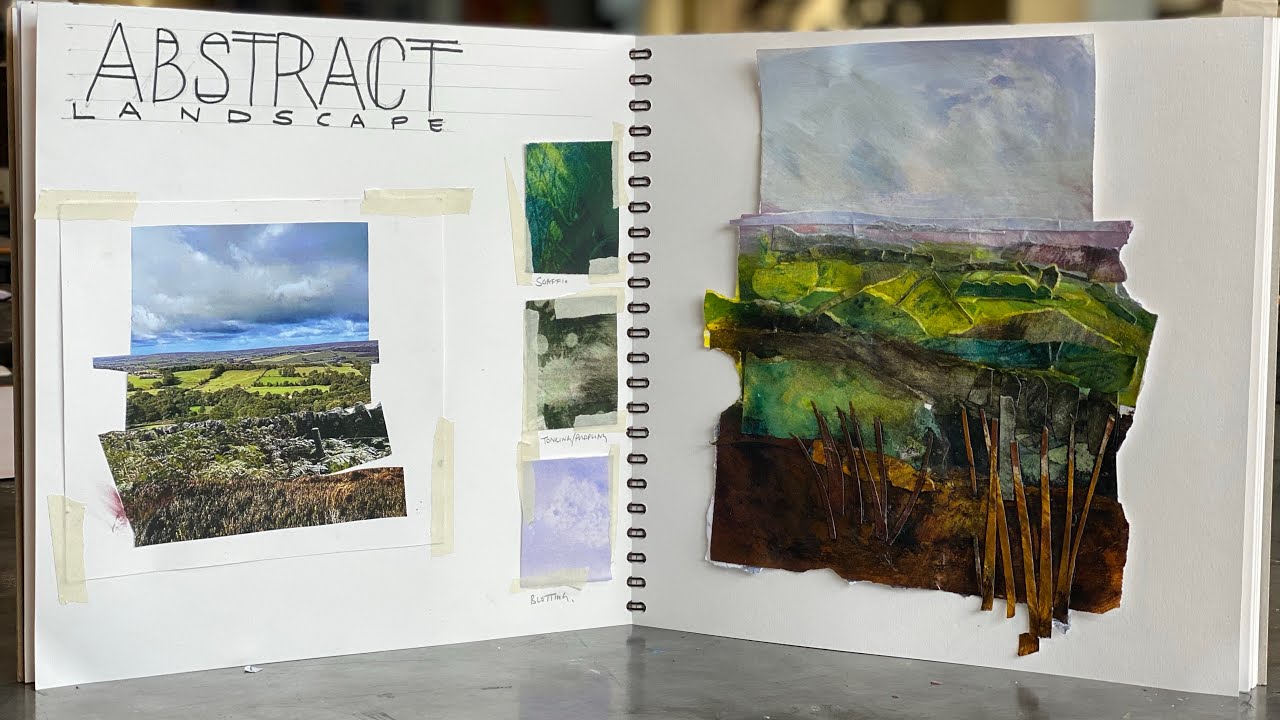The image is a horizontally rectangular, full-color photograph depicting an open spiral-bound book standing upright on a shiny, dark gray table, reflecting part of the book. The book's left page, prominently titled "Abstract Landscape" in black marker with artistic horizontal and vertical lines embellishing some of the letters, features a collage of landscape photographs. The topmost photo showcases a blue sky with white fluffy clouds. Below it, an aerial view of vast, green fields with scattered trees and rocks, culminating in a photograph of brown grass or wheat. Additionally, the left page is adorned with three smaller, taped-on pictures: a vibrant green scenery, a grayscale image with white spots, and another sky shot with a hint of blue and white. The right page diverges into an artistic rendition resembling the collaged photographs on the left. At the top, a painted blue and white sky looms over cliffs and green fields. Towards the bottom, the colors darken, transitioning to browns and dark greens, culminating in a depiction of dirt or stone at the base, punctuated by vertical spikes, all contributing to a cohesive representation of an abstract landscape.